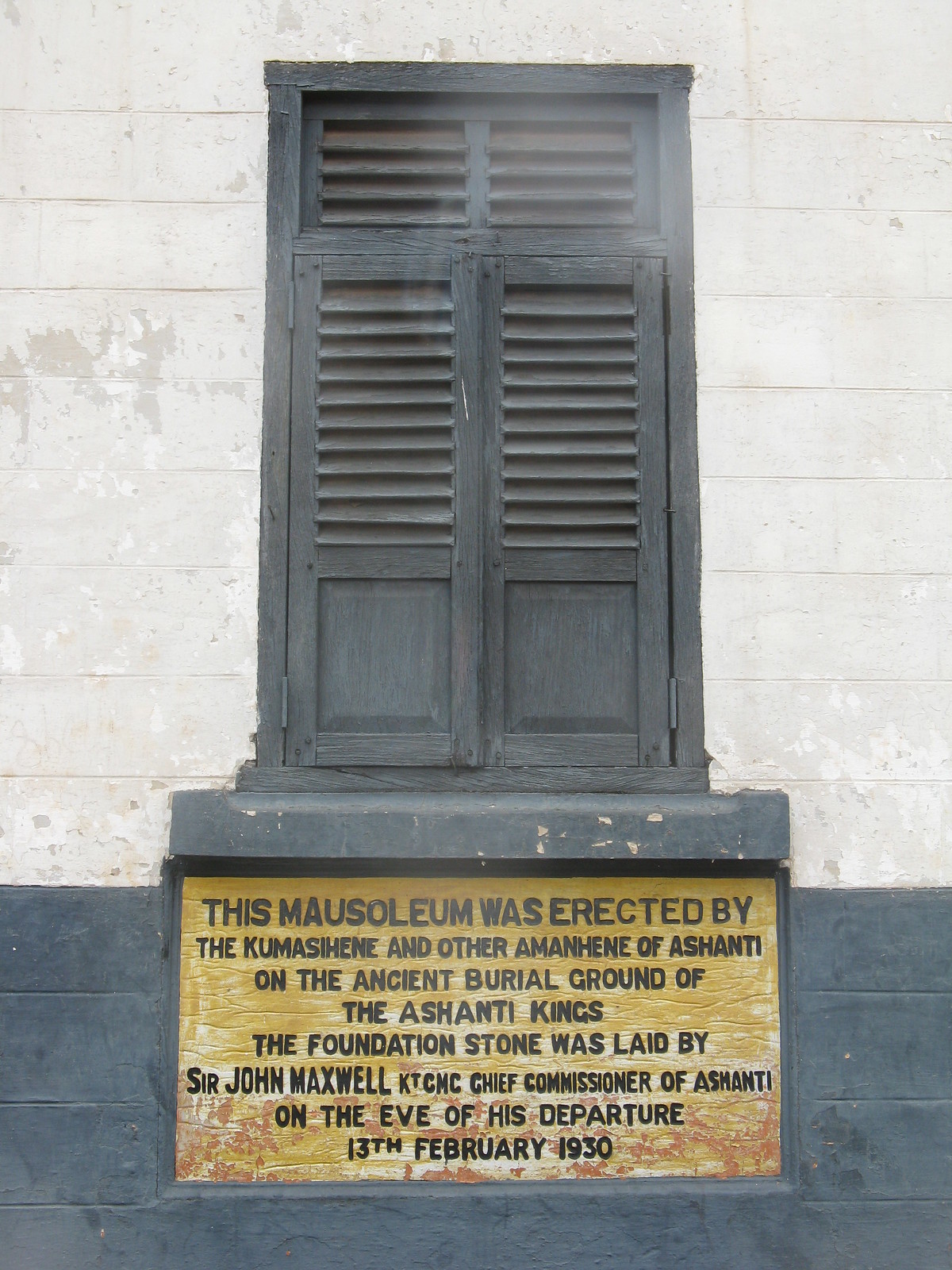A detailed photograph captures the entrance to a mausoleum, distinguished by its unique shutter-like charcoal gray double doors with slats extending halfway down, transitioning to a solid panel. The mausoleum is embedded within an aged white and gray brick wall, displaying a worn texture that adds a sense of history to the scene. The structure stands against a light cement concrete backdrop. Below the doorway, a weathered sign with a gold background and dark lettering bears significant historical inscriptions. The text reads: "This mausoleum was erected by the Kumashiren and other Amanhene of Ashanti on the ancient burial ground of the Ashanti kings. The foundation stone was laid by Sir John Maxwell, K.T.C., M.C., Chief Commissioner of Ashanti, on the eve of his departure, 13th February 1930." The upper portion of the sign shows more wear, revealing an orange and red hue, suggesting the passage of time.